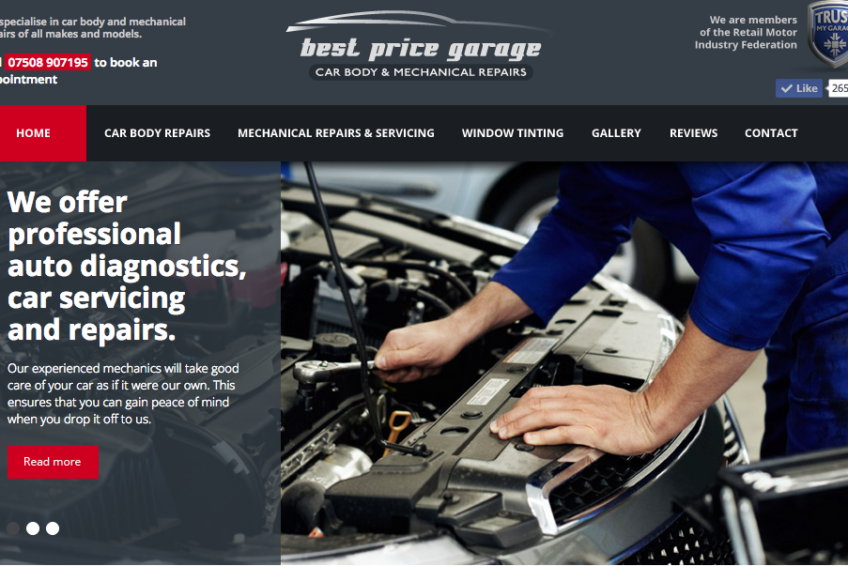This horizontal image represents a web page that could be accessed on a computer or smartphone. The background features a gradient of gray at the top. In the upper left corner, the text mentions a specialization in art, car body, and mechanical work. The sentence is partially cut off, but refers to services for all makes and models of vehicles. Next to this text is a red box with white numbers listing a phone number for booking appointments.

Centrally positioned are a couple of white lines separating sections of the page. Above these lines, the text reads "Best Price Garage," with "Car Body and Mechanical Repairs" stated underneath. 

In the upper right corner, there are small icons indicating memberships and engagement options. The icons signify trust by stating "We are members of the Retail Motor Industry Federation," along with "like" and "share" buttons for social media interaction. 

On the left side of the page, a navigation menu is displayed. The "Home" button is highlighted in red, whereas other menu options—such as "Car Body Repairs," "Mechanical Repairs and Services," "Window Tinting," "Gallery," "Reviews," and "Contact"—are shown in white text on a black background.

A visible portion of an image shows a person in a blue jumpsuit working on a car engine, with only their hands visible. To the left of this image, white text conveys that the garage offers professional auto diagnostics, car servicing, and repairs. It highlights the experience of their mechanics and indicates a link to "read more."